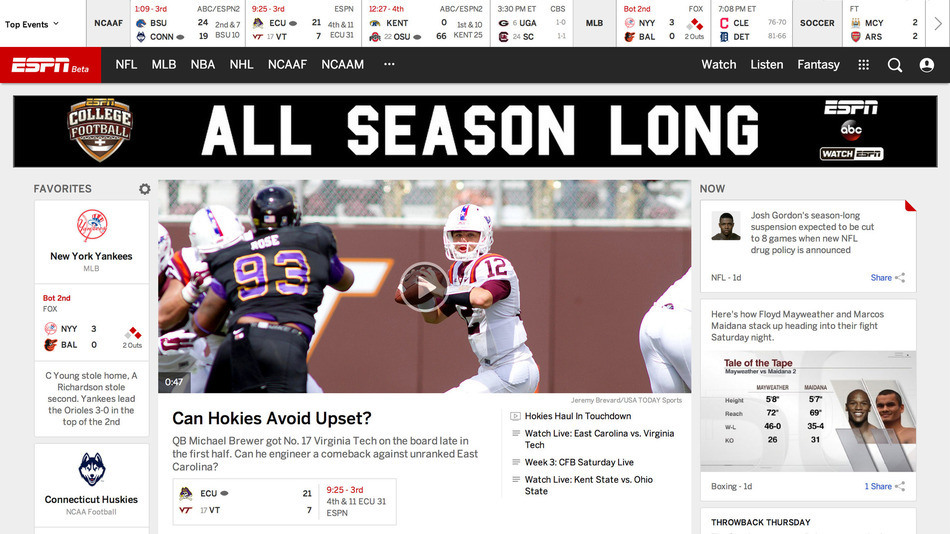The screen image displays the ESPN website homepage, prominently featuring the latest updates and scores for various sports. At the top, a highlighted section showcases the top events for NCAA Football (NCAAF), listing active and upcoming games, with some entries displaying live scores. Alongside NCAAF, updates are also available for Major League Baseball (MLB) and soccer.

A comprehensive toolbar beneath the main header allows easy navigation through different sports categories including NFL, MLB, NBA, NHL, NCAAF, and NCAAM. Additional options for watching, listening, and participating in fantasy sports are also accessible here.

Just below the navigation bar, a bold banner with a black background and white text declares, "All Season Long." This is followed by a summary of a recent New York Yankees game and a featured video of a freshly played football match. To the right, there are advertisements: one announcing that Josh Gordon’s season-long suspension is expected to be reduced to eight games under a new NFL drug policy, and another promoting a feature titled "Tale of the Tate."